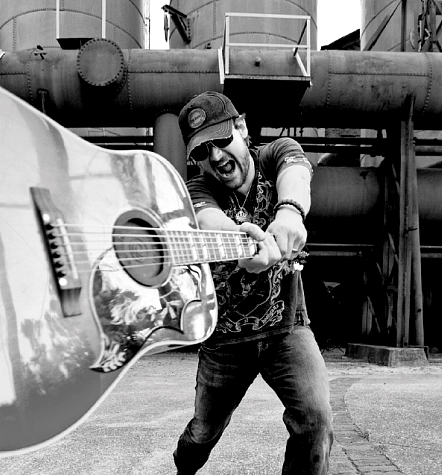In this black and white photograph, a man stands on concrete in what appears to be an industrial area, characterized by large pipes and storage tanks in the background. He is captured mid-motion, his mouth open as if screaming, and he's aggressively swinging a shiny, ornately designed, classic country-style guitar toward the camera. The reflection on the guitar suggests the presence of plants or foliage nearby. The man wears a dark cap with an indistinct logo, black sunglasses, a dark shirt adorned with lighter patterns, and jeans. His beard and mustache are closely trimmed. The setting is outdoors, with a partial view of the sky that appears clear, although the monochrome filter makes it difficult to determine cloud cover.